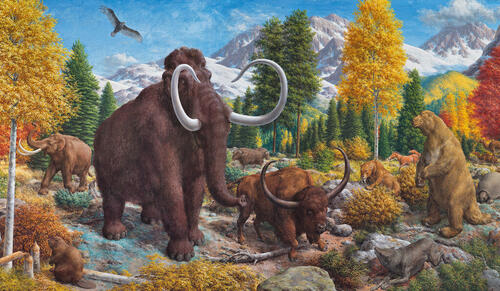This detailed painting showcases a vibrant scene set against a clear blue sky with wispy clouds that blend into the distant, snow-capped mountains. In the center, a large, brown woolly mammoth with gracefully curving white tusks stands prominently on rocky terrain. Just to its right, a smaller brown animal with horns—possibly a buffalo—faces in the same direction, adding depth to the scene. Nearby, a grayish animal, its identity obscured, appears at the lower right corner, where a brown bear stands upright on its hind legs, surveying its surroundings.

In the backdrop, lush autumn foliage presents a colorful tapestry of yellow, orange, and red, mingling with green pine trees. Among these trees, another mammoth—light gray and less woolly—can be seen, accompanied by other indistinct animals blending into the background. To the far left, a tall tree with yellow leaves stretches out of the frame while yellow bushes scatter near the base, adding to the scene's rich colors.

Overhead, a gray and black bird soars, its wings outstretched against the sky, while the rugged, snow-covered mountain range recedes into the distance, topping off this majestic tableau of ancient wildlife in their natural habitat.